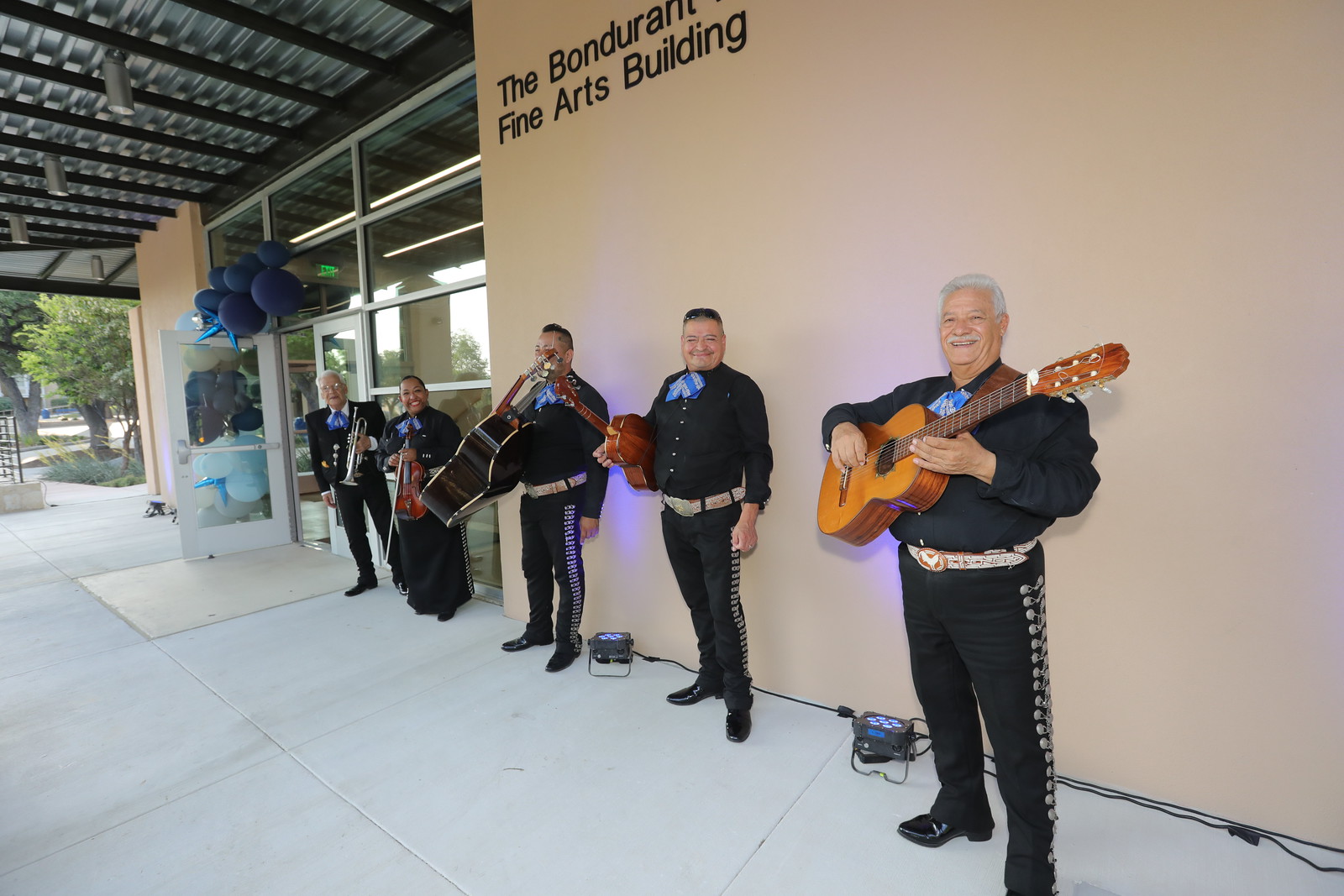In the vibrant outdoor setting of the Bondurant Fine Arts Building on what seems to be a sunny, celebratory day, a lively mariachi band stands in front of the building’s pinkish-beige wall. The entrance, adorned with large blue balloons, hints at a festive occasion, possibly a celebration of Fine Arts. The band is composed of five enthusiastic members, each dressed in strikingly coordinated mariachi attire: black shirts with blue and white bow ties, black pants with white ribbed sides, and black boots. Their diverse instruments—an acoustic guitar, a bass, a trumpet, a violin, and a trombone—indicate a rich, multicultural performance. The joyful expressions of the musicians signal their excitement and pride in showcasing their artistic talents. Framed by trees and grass in the background, the scene is further enhanced by lights on the ground, suggesting the potential for an equally enchanting evening show. The overall atmosphere exudes a charming, collegiate ambiance perfect for celebrating the arts.